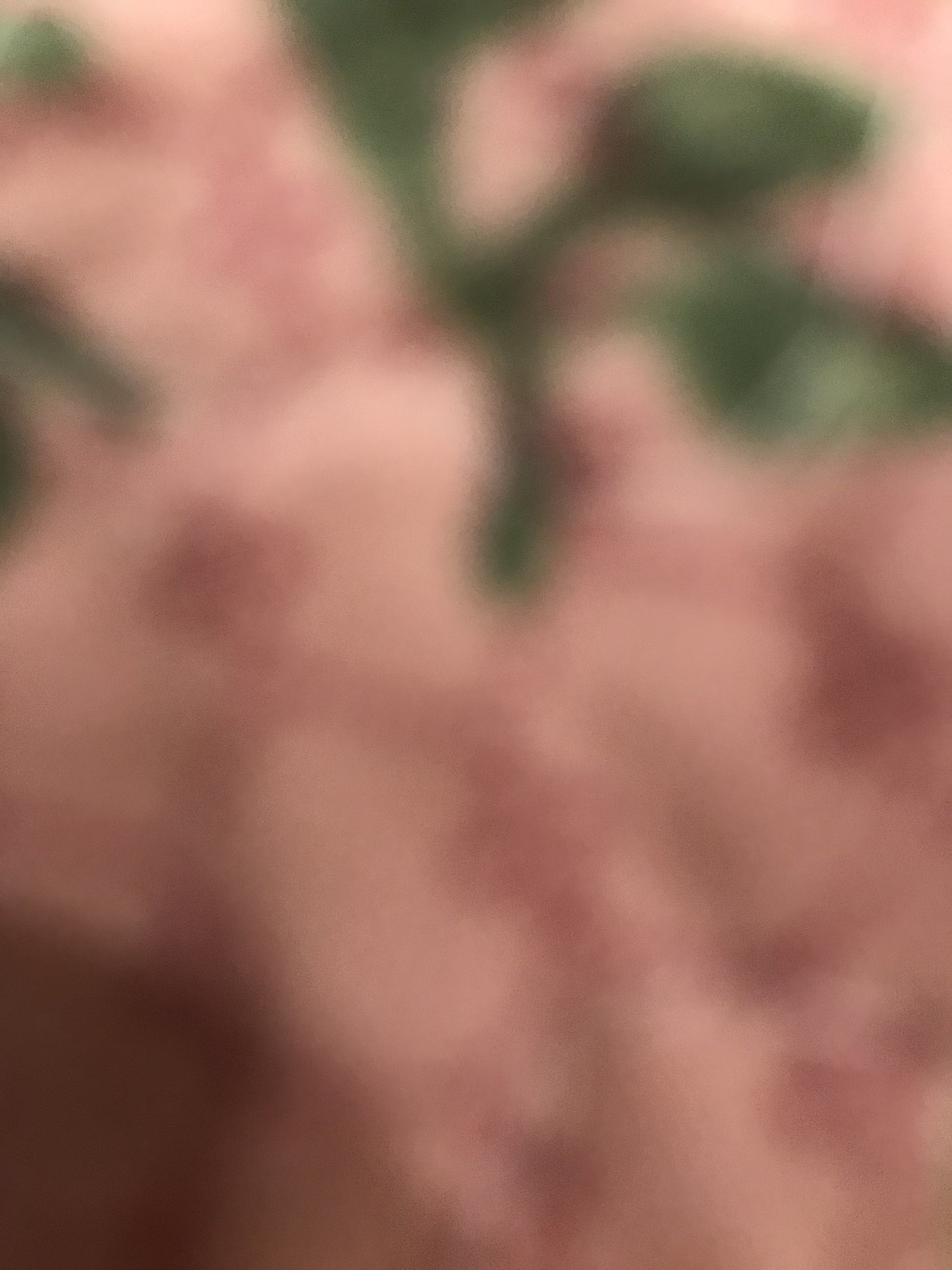The image is an incredibly blurry close-up shot of a surface with predominant pink tones. The lower left-hand corner is very dark, almost purple, while the majority of the image displays light pink hues. Dark pink and purplish lines create a rounded, swirling pattern throughout. In the upper half, amidst the pink areas, green lines appear, transitioning into green circular shapes in the upper right-hand corner, with shades varying from dark to medium to light green. The right side also shows a progression from darker brown at the bottom to a skin-tone-like color above. Despite the blur, the image gives an abstract, almost spray-painted look, merging the hues into an unintelligible but intriguingly patterned surface.